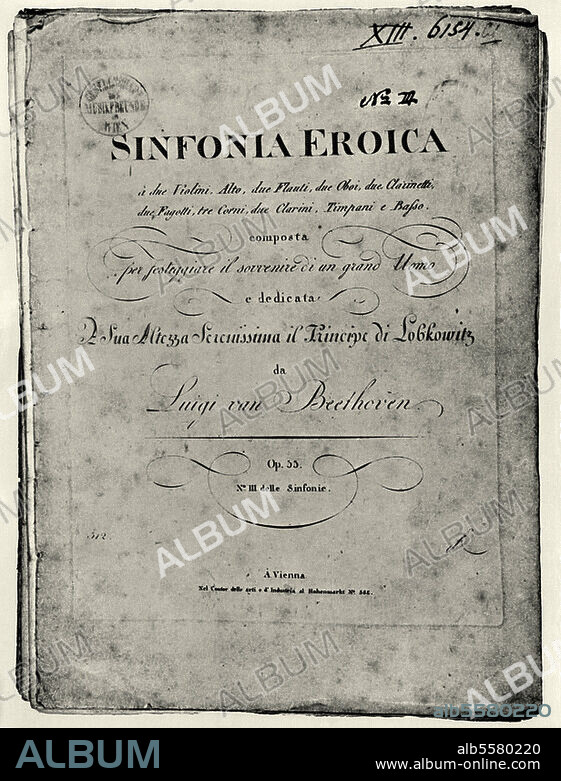The image appears to be of an album cover that has an ancient, historical feel, as if it were on a piece of parchment from the 1800s. The cover, which looks like a photocopy or scanned image, is heavily tattered and worn, featuring black and white hues with noticeable dirt and damage. Prominently displayed in the top middle of the cover is the title "Sinfonia Eroica" in bold font, surrounded by watermarks reading "album." Below the title, there's smaller cursive text and a line underneath stating "Luigi van Beethoven." The image also features additional text in a foreign, possibly Latin, language which is difficult to discern due to its faded and cursive nature. In the top left corner, a blurry, circular stamp hints at the origin of the document, while a black banner at the bottom of the image reads "album" on the left and "www.album-online.com" on the right. The cover overall has a gothic aesthetic with a sense of age and historical significance.